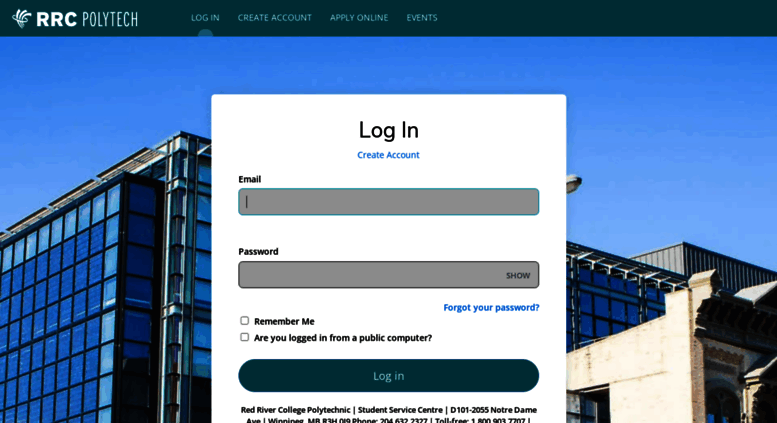This image depicts a web page for RRC Polytech, featuring a login section. At the top of the page, a green header prominently displays the "RRC Polytech" logo. Next to the logo, there are several navigation buttons: "Login," "Create Account," "Apply Online," and "Events."

Below the header, an image showcases a large modern building with numerous glass windows set against a bright blue sky. Overlaid on this image is a pop-up box for user login. The pop-up box is labeled "Login" at the top, followed by an option to "Create Account."

The login interface includes a field for "Email" with a corresponding typable box, followed by a "Password" field, also featuring a typable box. Below the password field, there are options to check "Remember Me" and "Are you logged in from a public computer?" Additionally, there is a "Forgot your password?" link beneath the password field.

At the bottom of the pop-up box, a green "Login" button is prominently displayed. Below this button, the text reads "Red River College Polytechnic Student Service Center."